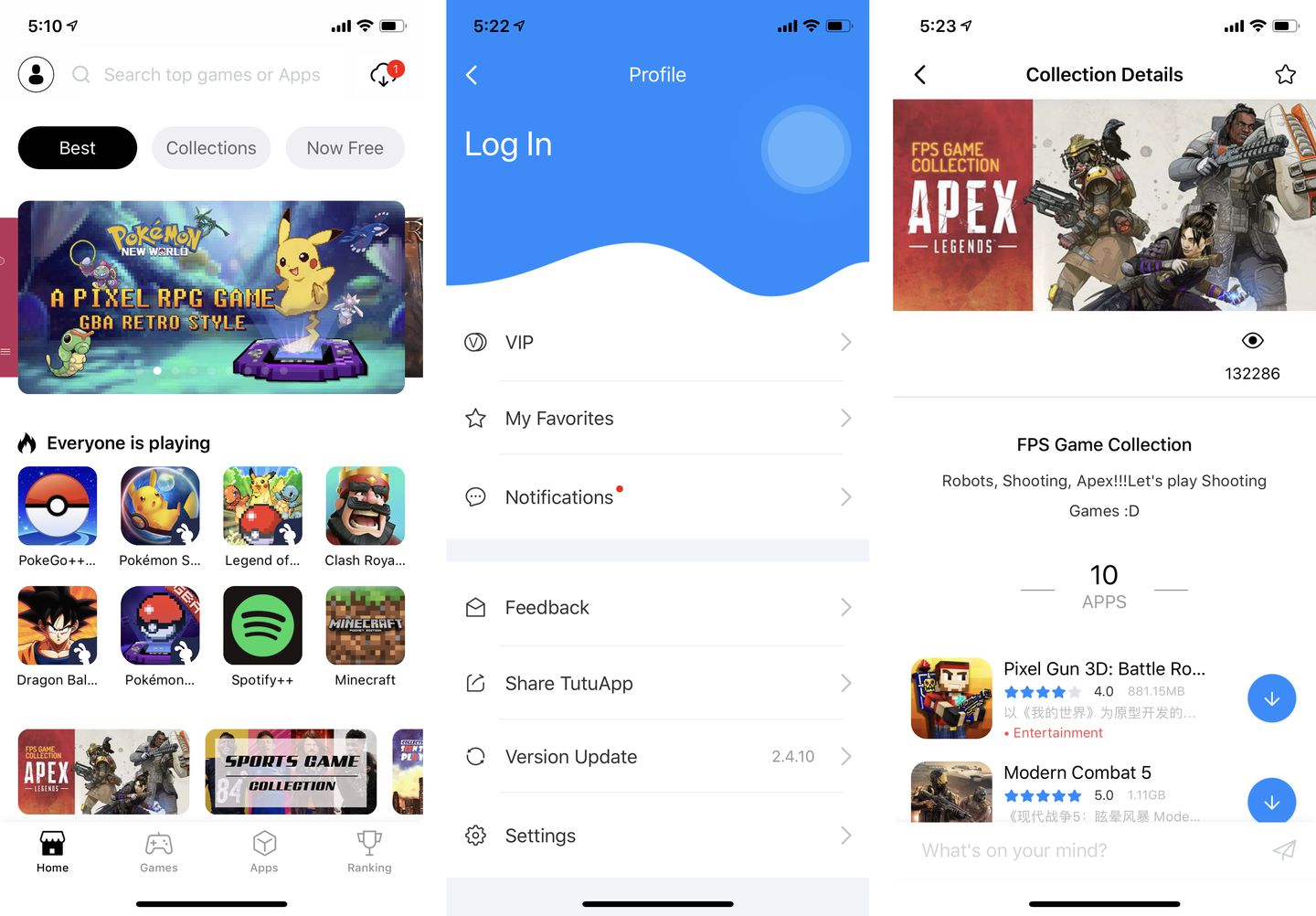Here are three sequential screen captures from a smartphone, possibly related to gaming applications. The first screen displays a pixelated RPG game reminiscent of Pokémon in a retro style. The caption reads, "Everyone is playing these games," likely indicating the popularity and widespread engagement with this genre.

The second screen capture is the profile login menu, showcasing several features for user customization and interaction. The visible options include "Profile Login," "VIP," "My Favorites," "Notifications," "Feedback," "Share To," "App Version," "Update," and "Settings." This screen allows users to personalize their gaming experience, stay updated, and connect with the wider community.

The third screen provides details about an FPS game collection, prominently featuring descriptions and themes of various first-person shooter games. The highlighted titles within this collection include "Apex Legends," characterized as a robot shooting game, and other shooting games. It further specifies that this collection contains 10 apps, with "Pixel Gun 3D" and "Modern Combat 5" being two examples available for download. These titles suggest a curated list of high-paced action games appealing to FPS enthusiasts.